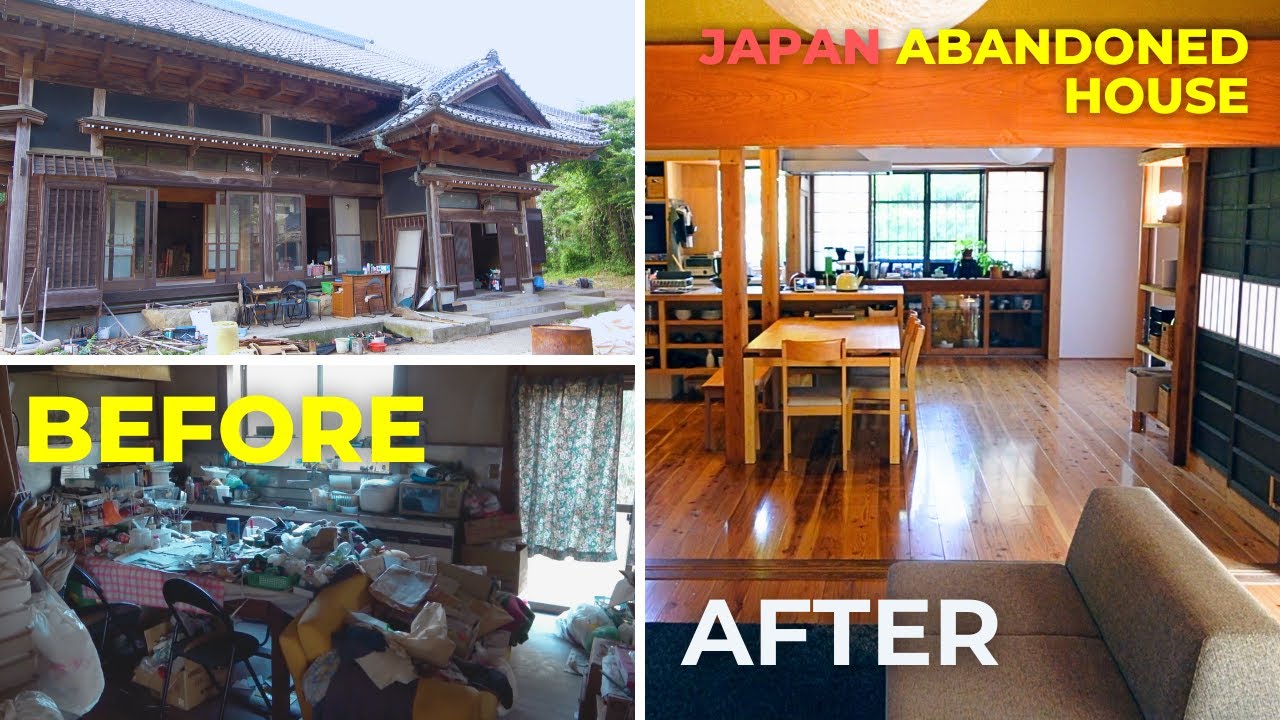This image is a striking before-and-after comparison of a renovated abandoned house in Japan. The top of the image is labeled "Japan Abandoned House," with "Before" written in bold yellow text over the left section and "After" in white on the right. The "Before" section shows two stacked images of the house in a state of disrepair. The exterior appears run-down with visible trash, debris, and open, dilapidated doors. Inside, the kitchen is cluttered with bags, food, and clothes scattered all over the table, counters, floor, and chairs. There is only a curtain serving as a makeshift door. In contrast, the "After" image displays a single, expansive view of the transformed interior. The space is now a clean, open-concept design featuring a shiny wooden floor, pristine white walls, and wooden accents. The table has been cleared, surrounded by wooden chairs and a bench. A chic gray couch and a blue rug enhance the modern aesthetic. Large windows at the back allow sunlight to flood in, illuminating plants on the kitchen counters and a cozy teapot or coffee pot on the stove, completing the warm and inviting ambiance.